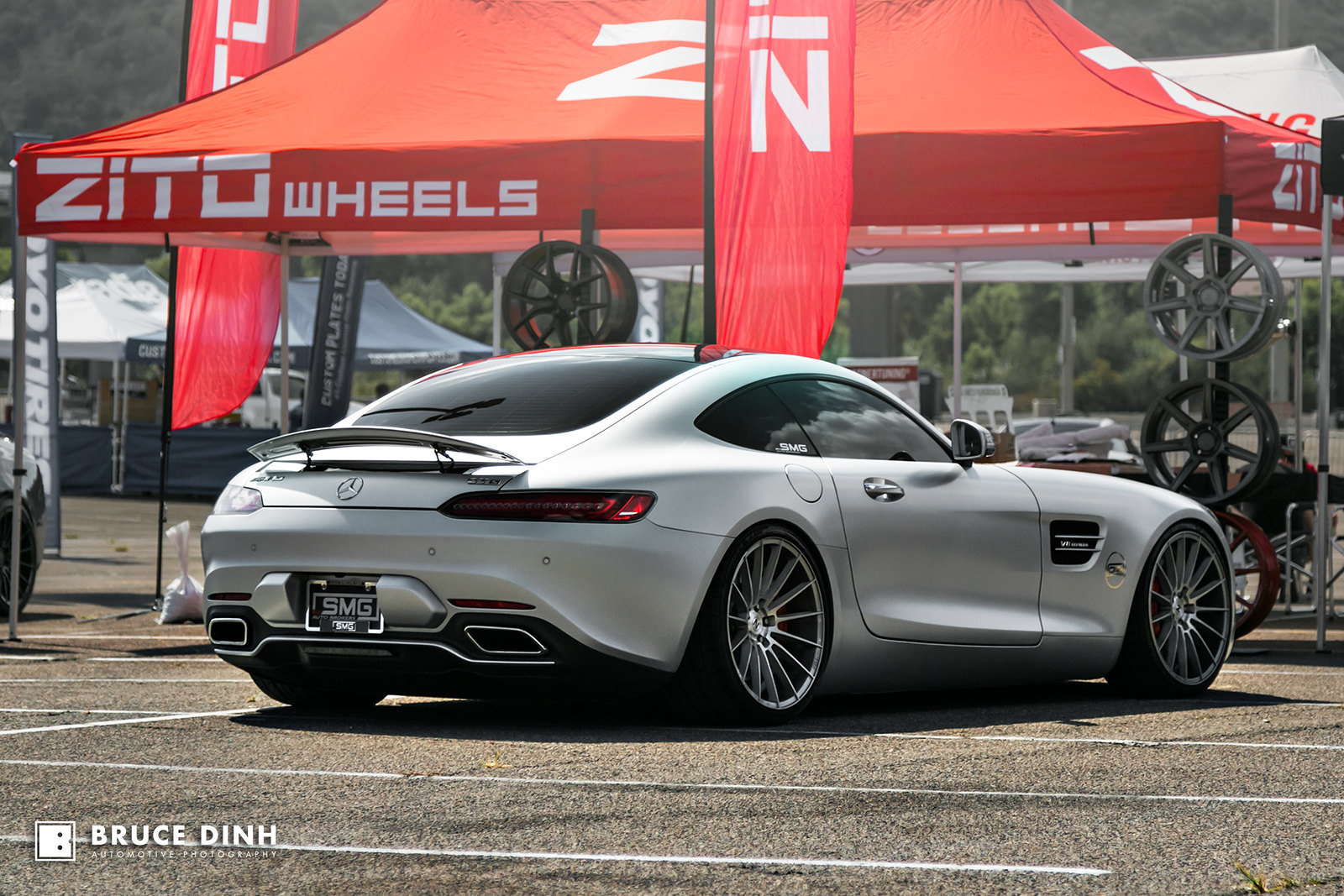The image captures a scene set in the middle of the day, likely at a car show. Centered in the image is a silver Mercedes sports coupe, parked diagonally on a gray asphalt parking lot marked with white lines. The car features fancy silver chrome wheels, a rounded back, an arched tail, and darkly tinted windows. Dominating the upper portion of the scene is a red pyramidal tent with white text that reads "Zito Wheels." Beneath this tent, several chrome wheels are neatly stacked. Additional red vertical banners and flags flutter around the tent. In the further background are more tents and a backdrop of green coniferous trees, enhancing the sense of an outdoor event. Visible colors in the image include gray, white, red, silver, orange, black, and green. The overall composition and setting suggest that this photograph was taken at a car show.